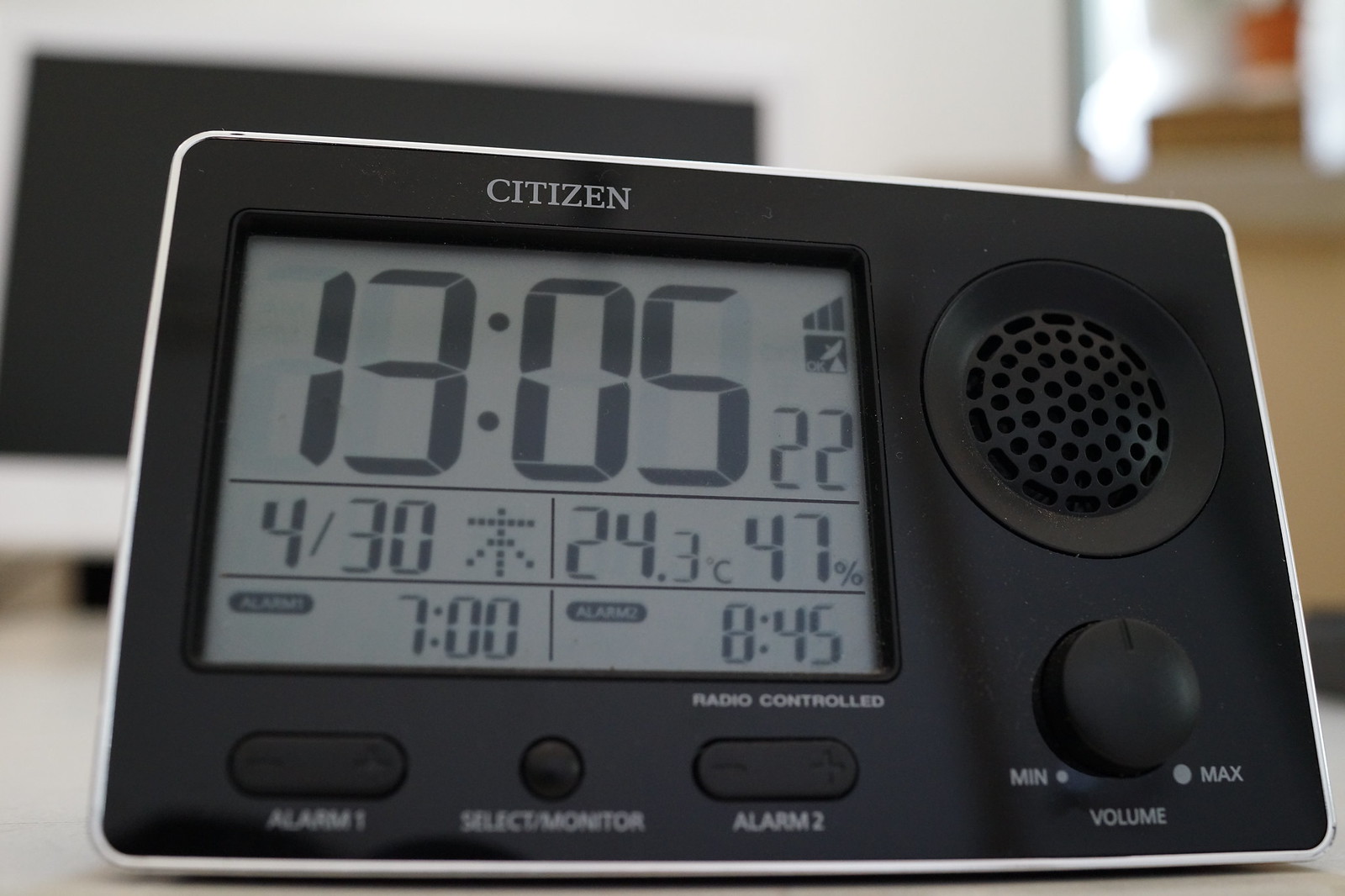A detailed close-up photograph showcases a black Citizen alarm clock, prominently featuring its digital display on the left side. Below the display are analog buttons for setting the alarm and adjusting the clock's settings. To the bottom right, a knob for volume adjustment is situated just below a small speaker. The brand name, "Citizen," is clearly visible on the upper-left side of the clock.

The digital screen reads a precise time of 13:05 and 22 seconds. The clock seems capable of receiving either satellite signals or FM/AM radio signals. Below the time, the display is divided into four distinct quadrants: the top left shows the date, "4.30," along with a kanji symbol. The upper right quadrant shows "24.3 degrees Celsius" and "47%," likely indicating temperature and humidity. The lower left quadrant displays two set alarms: Alarm 1 is set for 7:00 AM and Alarm 2 for 8:45 AM.

In the background, a TV display is blurred but discernible, with an off-white, cream-colored wall behind it. The top right section of the background hints at a hallway. The low-angle shot of the alarm clock gives the frame a slightly warped perspective, adding to the unique visual appeal of the image.